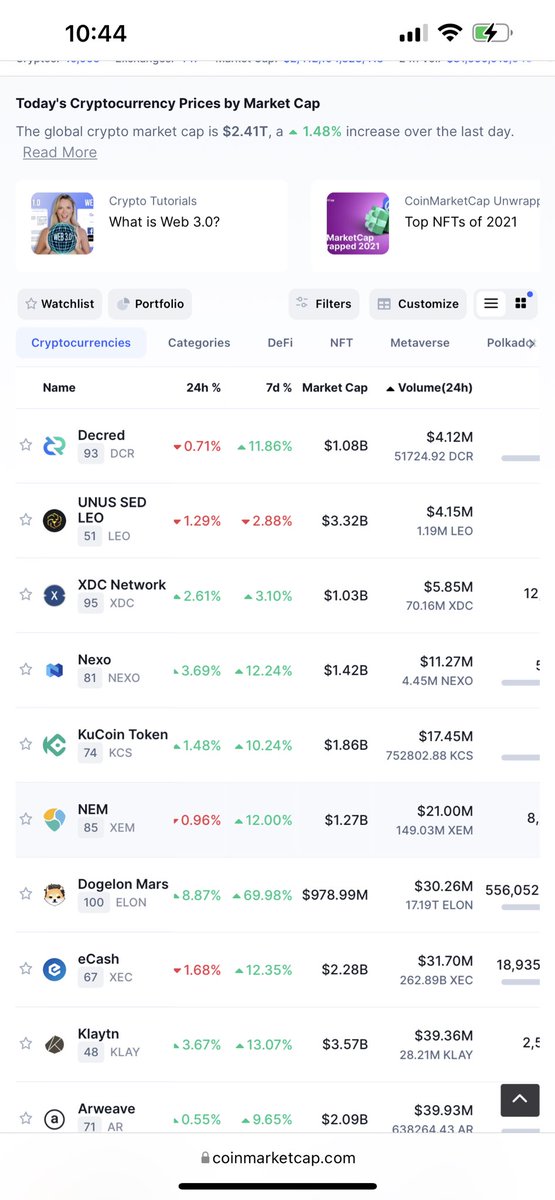**Detailed Caption:**

This image captures a screenshot from a mobile device displaying a cryptocurrency market update. The top part of the screen features common mobile indicators on a white background: '10:44 AM' is displayed in black on the left, while on the right, icons for mobile signal strength, Wi-Fi strength, and a half-charged battery appear in green and white. The main content presents "Today's cryptocurrency prices by market cap," indicating that the global crypto market cap is $2 trillion with a 1.48% increase over the last day. Below this, there is a user interface including a picture of a woman's head with the text "crypto tutorials," showing emphasis on educational content related to Web 3.0, positioned next to an image of a globe on a purple background with a caption "Coin Market Cap on wrap, top NFTs of 2021."

Further down, navigation buttons such as Watchlist, Portfolio, Filters, Customize, and Cryptocurrencies (which is highlighted in blue) are visible. A tabulated section categorizes cryptocurrencies into groups like DEFI, NFT, Metaverse, and Polkadot. Following this, a table lists various cryptocurrencies including Decred, Unisat, Leo, XDC Network, Nexo, KuCoin Token, NEM, Dogalon Mars, eCash, Kalato, and Armweave, displaying their 24-hour percentage changes—positive changes in green and negative changes in red—along with market cap values and volume percentages.

At the bottom center of the page, the secured website "Coinmarketcap.com" with a padlock icon is noted, underlined by a thin horizontal black line that spans across the page's width. A small black square with an up arrow is located in the right-hand corner, suggesting a jump-to-top function or sharing option. The detailed interface signifies comprehensive cryptocurrency market tracking and analysis.